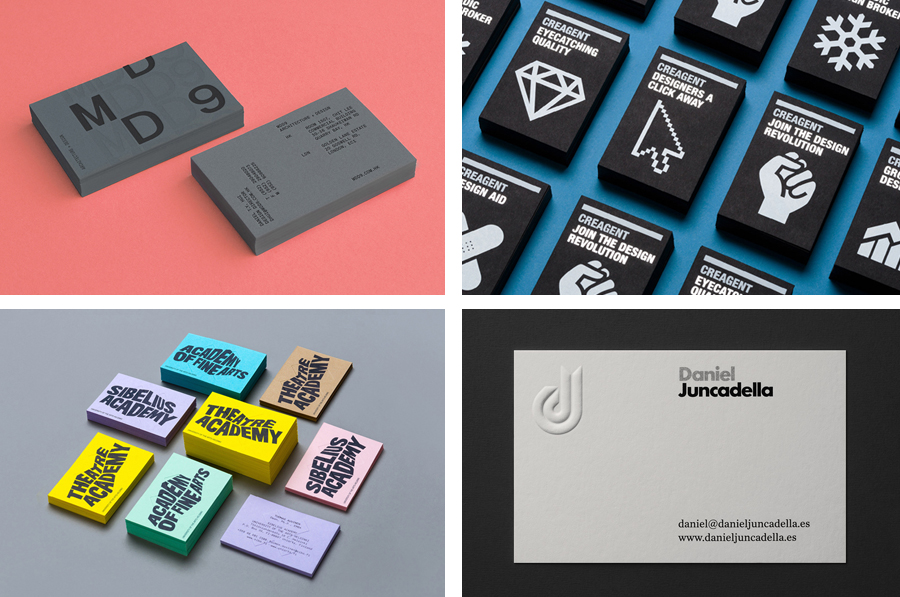The image is a composite of four distinct frames, each presenting a different type of printed material against varied backgrounds. 

The top left frame features a pink background adorned with two gray rectangles exhibiting black, illegible text, which may be business cards or informational slides. 

The top right frame showcases a blue background with a series of black rectangular prisms. Each prism contains white and gray text related to a design agency, identified as "Creagent." The texts read: "eye-catching quality" with a diamond icon, "designers a click away" accompanied by a pixelated white cursor, and "join the design revolution" next to a clenched fist. Multiple repetitions of these prisms are partially visible along the right edge. 

In the bottom left frame, a gray background presents a colorful array of stacked paper or business cards, in shades of blue, brown, purple, yellow, teal, pink, and lavender. Most of these stacks feature black, wavy text that reads "Theater Academy," while the lavender stack displays thin, black illegible text.

The bottom right frame contains a stark black background with a central white rectangle. The top left of this rectangle has an embossed "D" logo in white, alongside the name "Daniel" in gray text and "Junkadella" in black text below it. At the bottom right, contact details are provided: "Daniel at danieljunkadella.es" followed by "www.danieljunkadella.es."

The variety of business cards, promotional materials, and contact information suggests a comprehensive presentation of design and print capabilities.